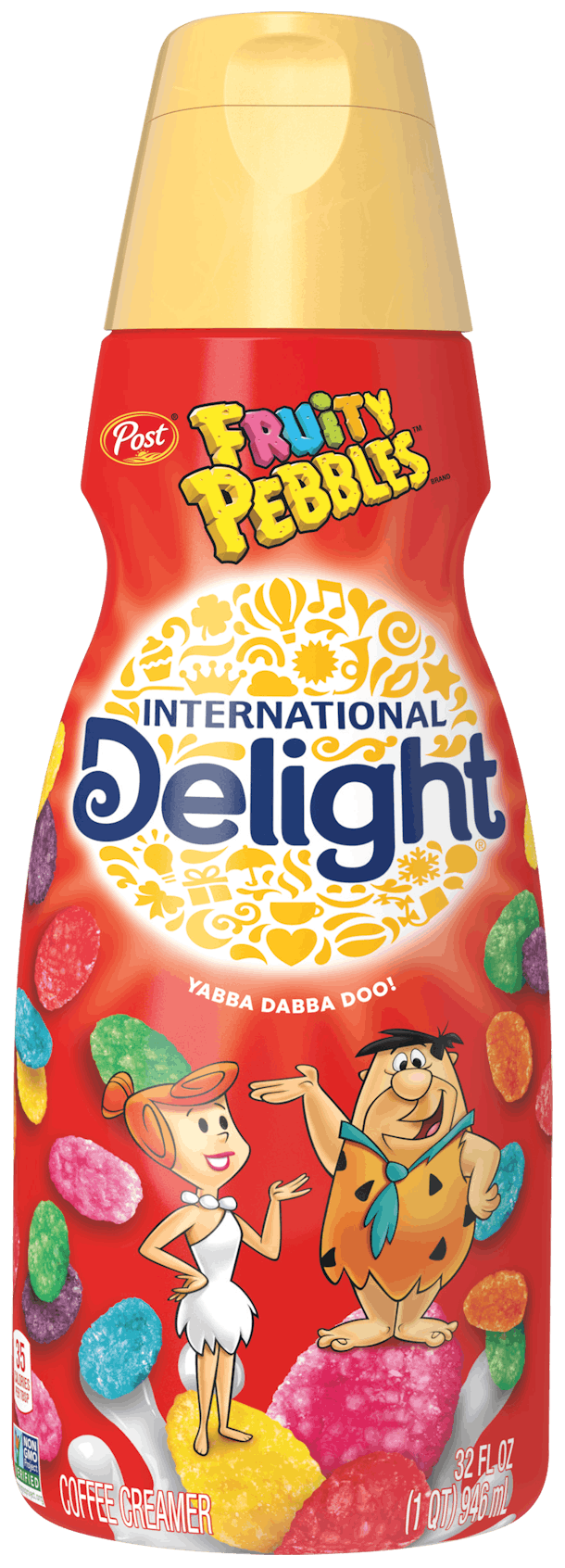The image showcases a zoomed-in, large bottle of Post Fruity Pebbles International Delight Coffee Creamer against a pure white background. The bottle prominently fills the entire frame and is centered perfectly, resembling an advertisement style. The bottom portion of the bottle is red, featuring the 'Post' logo in the upper left corner and the 'Fruity Pebbles' brand name in colorful, slanted text to the right. The upper portion includes a gold flip-top lid. A central white circular area adorns the bottle, embellished with gold shapes like music symbols, suns, and hearts. Positioned across this circle, the text 'International Delight' appears in blue. Below, in small white text, it reads 'Yabba Dabba Doo.' The bottle also features an illustration of Fred and Wilma Flintstone, each standing on colored Fruity Pebbles—Fred on a pink one and Wilma on a yellow one—with one hand on their hips and the other pointing towards each other. The label indicates the product is a 32 fluid ounce coffee creamer. The vibrant colors present include red, gold, white, yellow, pink, blue, green, and orange.